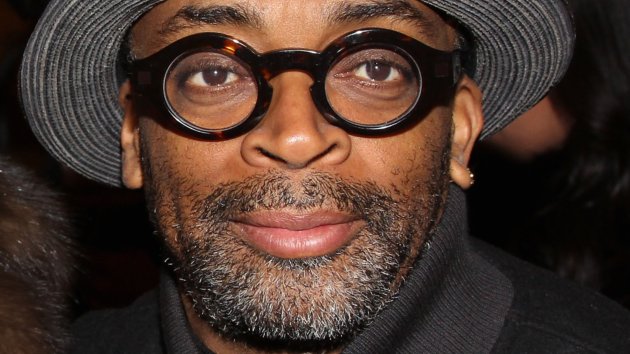The photograph is a close-up of an African-American man, prominently believed to be Spike Lee, the renowned director. He has rich, light brown skin and is sporting a black, salt-and-pepper beard and mustache. His facial hair hints at a combination of black, white, and gray, suggesting he may be in his 50s. He has a single earring in his right ear. His eyes are framed by distinctive, circular tortoise shell glasses that stand out against his dark eyebrows and brown eyes. He is wearing a black sweater with a gray turtleneck that reaches up to his ears, and possibly a black jacket over it. His head is adorned with a black woven hat with a brim that encircles it, noticeable for its unique white ringed rim, which contrasts with the dark background surrounding him. The setting appears blurred with an indistinct presence of a figure with black hair off to the right, emphasizing the focus on the man's contemplative expression.